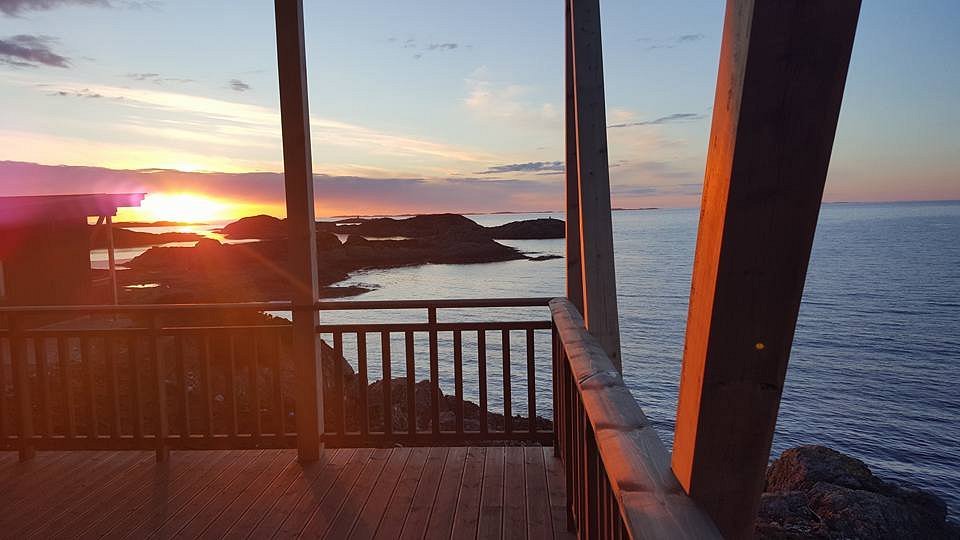The image captures a serene sunset over a tranquil ocean, taken from a wooden deck or patio of a house or resort condo. The ocean lies within a cove, bordered by a jagged, rocky shoreline with no signs of a sandy beach, just layers of rocks extending into the water. Smaller rocks also appear closer to the camera. The setting sun, positioned on the left side of the image, bathes the scene in a palette of yellow, orange, violet, and blue hues, transitioning to a deeper blue as it nears the camera. Dark clouds hover directly above the sun, casting a striking contrast with their black and deep purple colorations. The horizon remains flat, emphasizing the calmness of the water, which displays gentle ripples and distant landmasses visible only by their silhouettes. The scene exudes a natural beauty, capturing the peaceful essence of nature just as day turns to dusk.